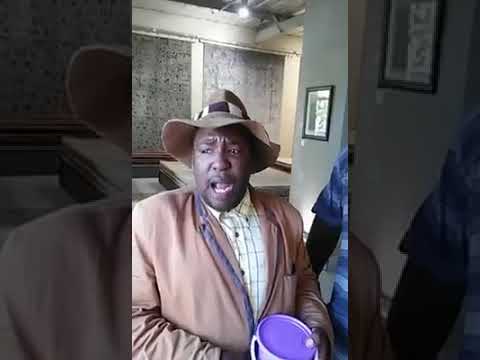The image features two black men positioned against a partially decorated background consisting of a white wall with brown floral curtains and a column with framed pictures. The man on the left is wearing a brown hat with a black-and-white ribbon, a light brown jacket over a yellow button-up shirt adorned with black lines in a tic-tac-toe pattern. He holds a pink container with a sloping white handle close to his stomach and has a slightly open mouth with a furrowed brow, gazing slightly to his right. The taller man on the right, dressed in a short-sleeved shirt with horizontal stripes in various shades of blue, including dark blue and light blue, is looking down to his left with a visible smile, revealing some teeth. His arm is positioned behind the shorter man's arm. The right side of the picture presents a close-up of the taller man’s face with his striped shirt, while the left side displays a close-up of the shorter man's left ear, part of his hat, and shoulder, along with the background tapestry.